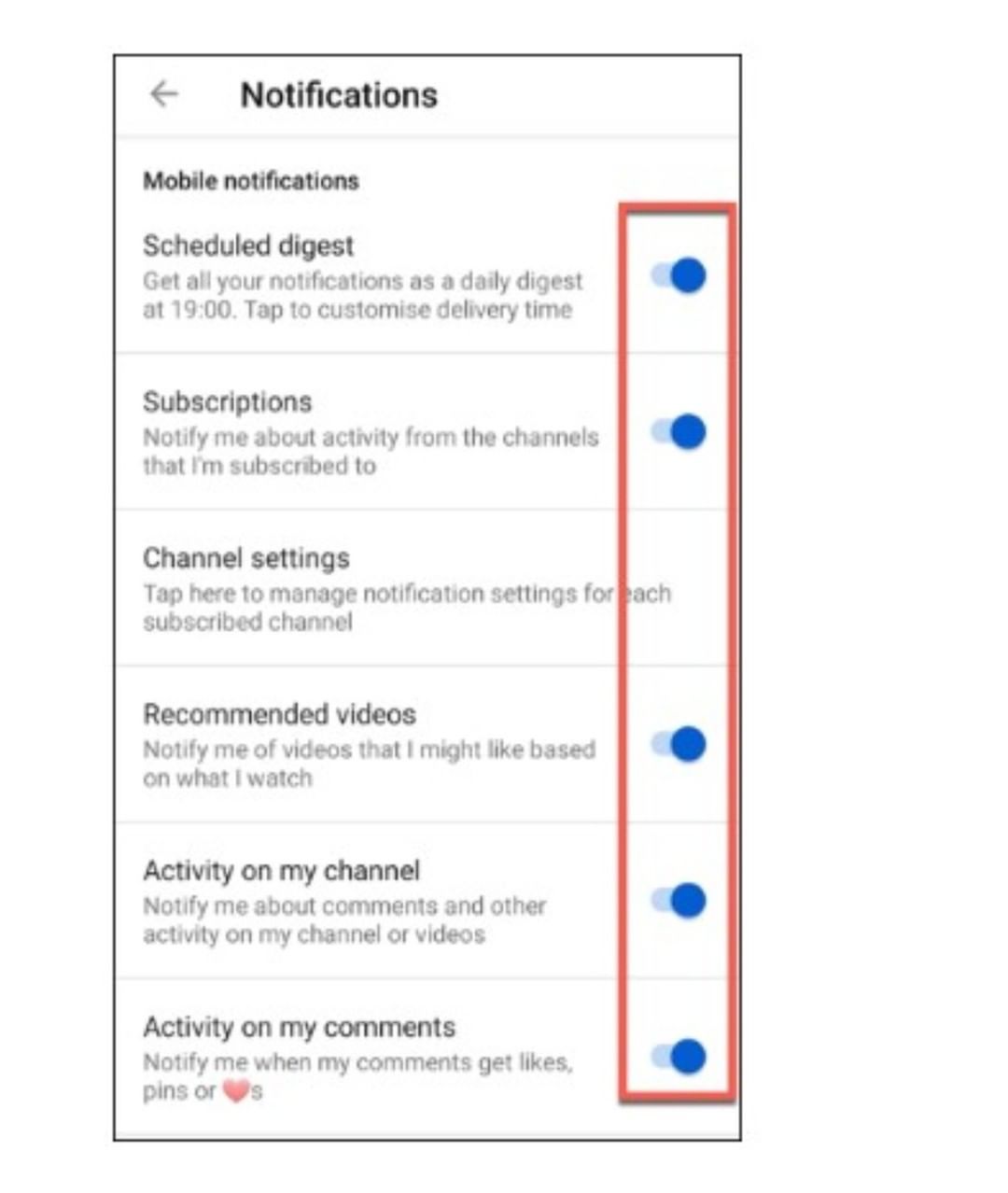Here is a cleaned-up and detailed caption for the image described:

"A screenshot of mobile notification settings on a smartphone is displayed. At the top of the screen, the title 'Notifications' is shown with a left-pointing arrow, indicating a way to navigate back to the previous menu. Below, in bold black font, it says 'Mobile Notifications.' 

The settings listed, each accompanied by a toggle switch, are as follows:

1. **Scheduled Digest**: This setting allows the user to receive notifications as a daily digest. The toggle switch is blue, indicating it is turned on.
2. **Subscriptions**: This setting notifies the user about activity from the channels they are subscribed to. It is also toggled on with a blue switch.
3. **Channel Settings**: This setting invites the user to tap and manage notification settings for each subscribed channel. Notably, this option does not include a toggle switch.
4. **Recommended Videos**: This setting sends notifications about videos that the user might like based on their viewing history. It is toggled on with a blue switch.
5. **Activity on My Channel**: This setting alerts the user about comments and other activities on their channel or videos. This is toggled on with a blue switch.
6. **Activity on My Comments**: This setting notifies the user when their comments receive likes, pins, or hearts. It is toggled on, as indicated by the blue switch. For this setting, a red heart icon followed by the letter 's' is used to indicate 'hearts.'

All the toggle buttons are highlighted within a red rectangular border."

This detailed caption provides a clear and comprehensive understanding of the screenshot of the notification settings.